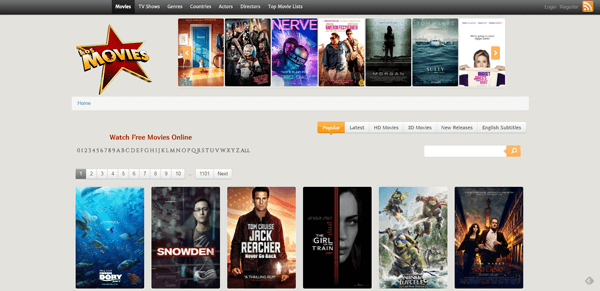This image depicts a screenshot from a movie rental or free movie streaming platform. Dominating the top section of the interface is a vibrant red star with a gold outline, prominently displaying the word "Movies" at its center. Above this, a navigation menu offers various categories including "Movies," "TV Shows," "Genres," "Actors," and "Top Movie Lists" or possibly "Blockbusters," though the latter is somewhat unclear.

Below the navigation bar, a selection of movie posters is displayed in a grid format. Among the titles visible are "Nerve," "Finding Dory," "Snowden," "Jack Reacher," "The Girl on the Train," and "Teenage Mutant Ninja Turtles." There are also several other indistinct titles.

Towards the bottom of the screen, options are available to help users filter the movie collection. Sorting options include categories such as "Popular," "Latest," "3D Movies," "New Releases," and "English Subtitles," suggesting a user-friendly interface designed to enhance the movie-watching experience.